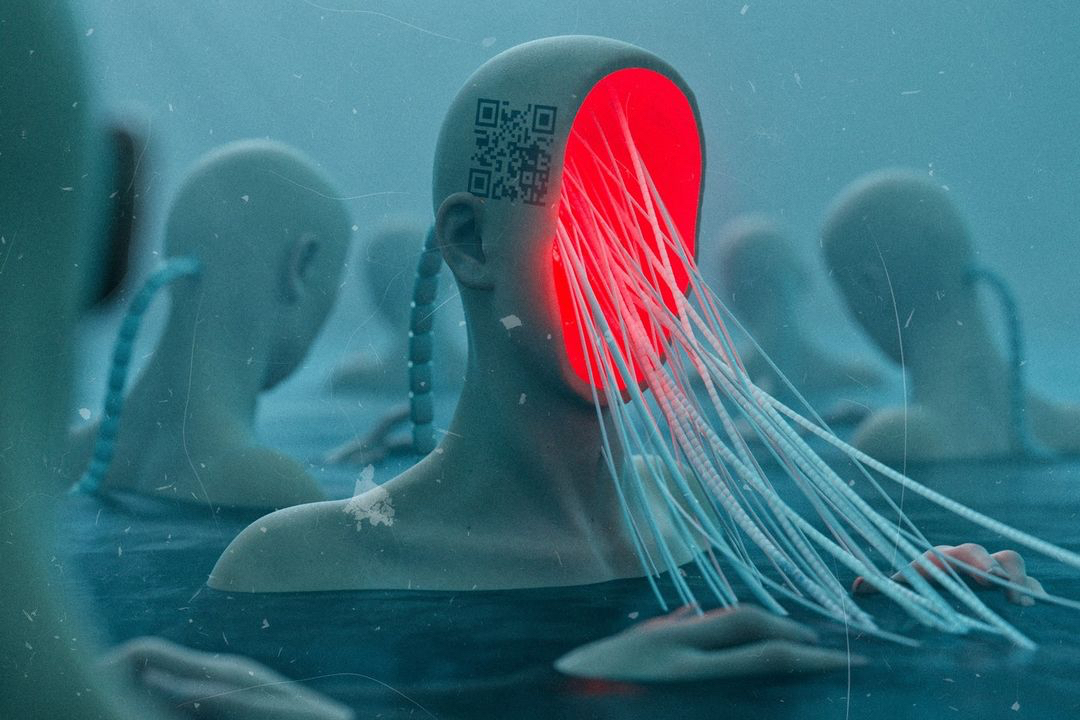The image is a surreal, rectangular illustration dominated by blue hues, depicting multiple mannequin heads and shoulders immersed in water up to their collarbones. The central mannequin, serving as the focal point, features an eerie, glowing red-pink oval where its face should be. Emerging from this illuminated area are long, white strands that reach down into the water, where disembodied hands with visible fingertips float near the surface. Additional details include a QR code on the side of the central mannequin's head and cords protruding from the back of each mannequin's neck. The other mannequins are positioned facing away, presenting featureless, flat surfaces instead of faces. The background remains consistently blue, enhancing the otherworldly atmosphere of the scene.